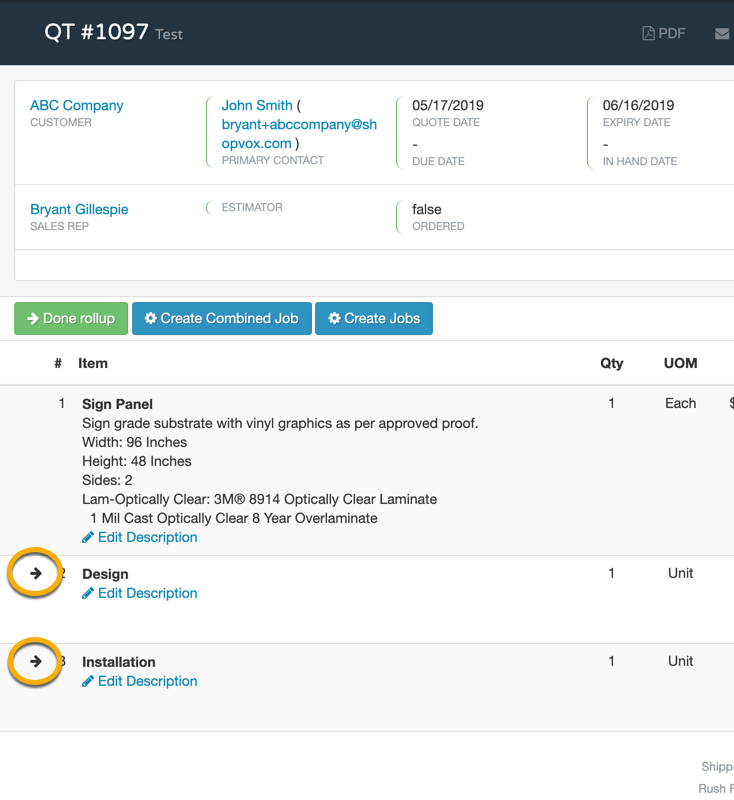This detailed caption effectively captures the layout and contents of the website displayed in the image. Here is a cleaned-up, descriptive version:

---

The image displays a detailed view of a website interface. In the top left-hand corner, there is a rectangular black bar. Inside this bar, from left to right, it reads "QT" in white, followed by "#1097" in white, and "test" in light gray. On the far right of this bar, it mentions "PDF" in light gray, accompanied by an envelope icon.

Below this, on the left side of the screen, the background is gray with a horizontal white rectangle inside. In the top left of this rectangle, it says "ABC Company" in white, and beneath it, in blue, it reads "Customer" with the name "John Smith, Bryant" followed by an email "ABCCompany@shopvox.com." Underneath, "Primary Contact" is displayed in light gray.

To the right, another section mentions "5-17-2019" in black as the quote date, with "Quote Date" in gray below it. Additionally, a minus sign in black followed by "Due Date" in gray is listed. Further right, the "Expiry Date" shows "6-16-2019" in black, with another gray minus sign below, labeled "In Hand Date."

Further down on the left, "Brian Gillespie" appears in blue with "Sales Rep" in gray beneath. To the right, "Estimator" is in gray, and "False" is in black with "Ordered" in gray underneath.

Continuing downwards, there are several buttons. On the left, a green button with a right-facing arrow says "Done Roll-up." Next to it, moving right, a blue button with white text states "Create Combined Job," followed by another blue button saying "Create Jobs" in white.

Below these, a table begins. On the left, a black number sign is followed by "Item" in black. To the far right, "QTY" and "UOM" are listed in black. Under these headings, the number "1" aligns below the number sign. For "Item," it lists "Sign Panel" in black, detailing specifications such as "sign grade substrate with vinyl graphics as per approved proof, width 96 inches, height 48 inches, sides 2, LAM — optically clear 3M, 8914 optically clear laminate, 1MIL cast optically clear 8-year over laminate." To the right, under "Quantity," it states "1," and under "UOM," it reads "Each."

Further down, another orange circle with a right-pointing black arrow is labeled "Design" in bold black letters. Below, a pencil icon and blue text say "Edit Description." To the far right, it again lists "1" under "Quantity" and "Unit" under "UOM."

At the bottom-most bar, another orange circle with a right-facing black arrow is labeled "Installation" in black, with a pencil icon and "Edit Description" in blue beneath. Finally, to the right, it states "1" under "Quantity" and "Unit" under "UOM."

---

This rewritten caption meticulously describes the visual elements and textual information present on the website in a structured and detailed manner.